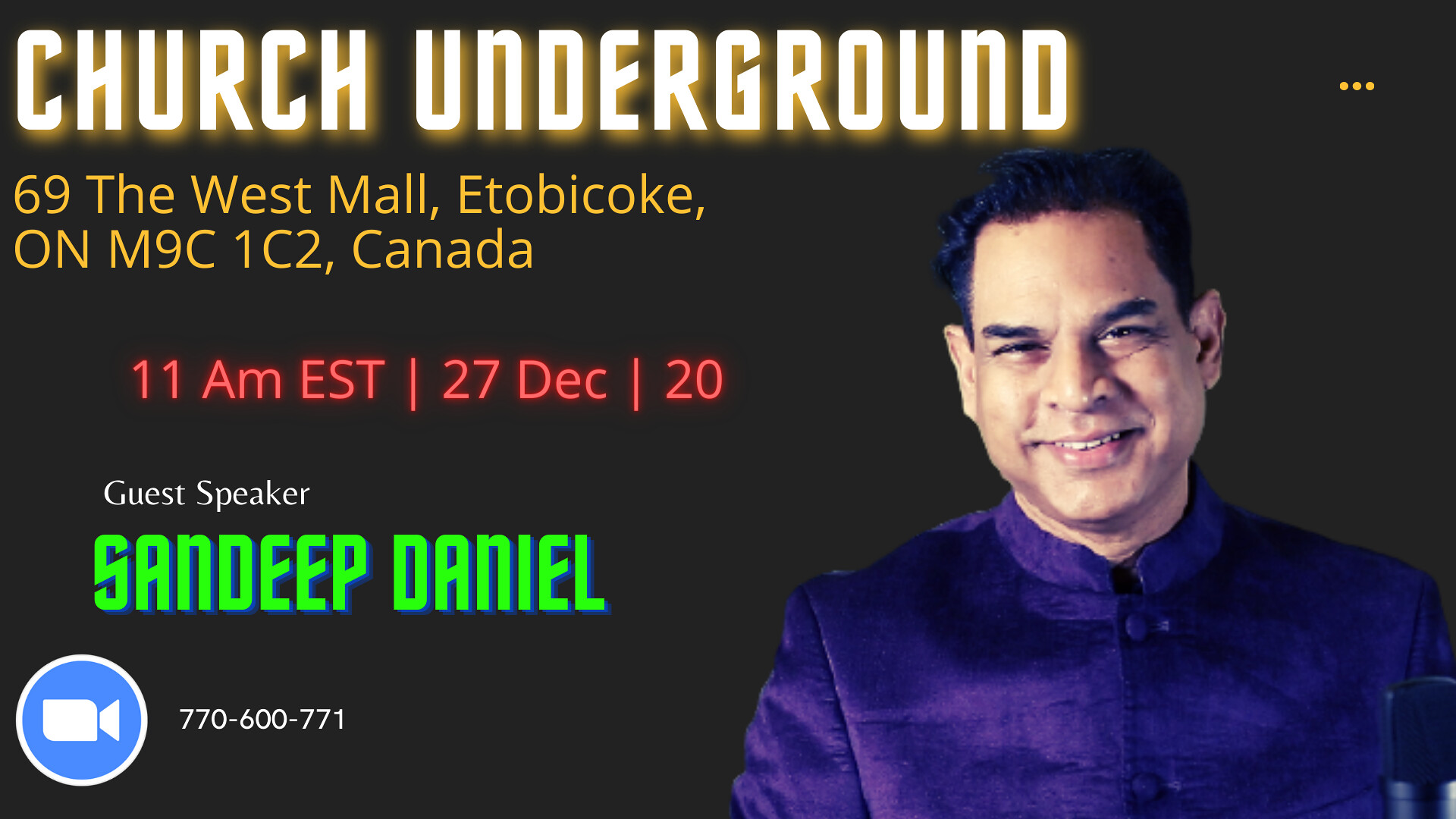The digital advertisement, set in landscape mode against a deep gray-black background, prominently displays "CHURCH UNDERGROUND" in bold white print with a yellow shadow effect in the top left corner. Beneath the headline, the address is listed in yellow: "69 The West Mall, Etobicoke, ON M9C 1C2, Canada." Below the address, in red text, the event's details read: "11 a.m. EST | 27 December | 20." The guest speaker, "Sandeep Daniel," is highlighted in large green print with a blue shadow effect, and the phrase "Guest Speaker" appears above his name in small white print. In the lower left corner, there is a blue circle enclosing a white video camera icon, next to which the contact number "770-600-771" appears. The upper right corner displays an ellipsis of three gold dots. On the right-hand side of the image, there is a clean-shaven man of Indian descent with short, black hair, smiling at the camera and wearing a blue-colored bandh gala.